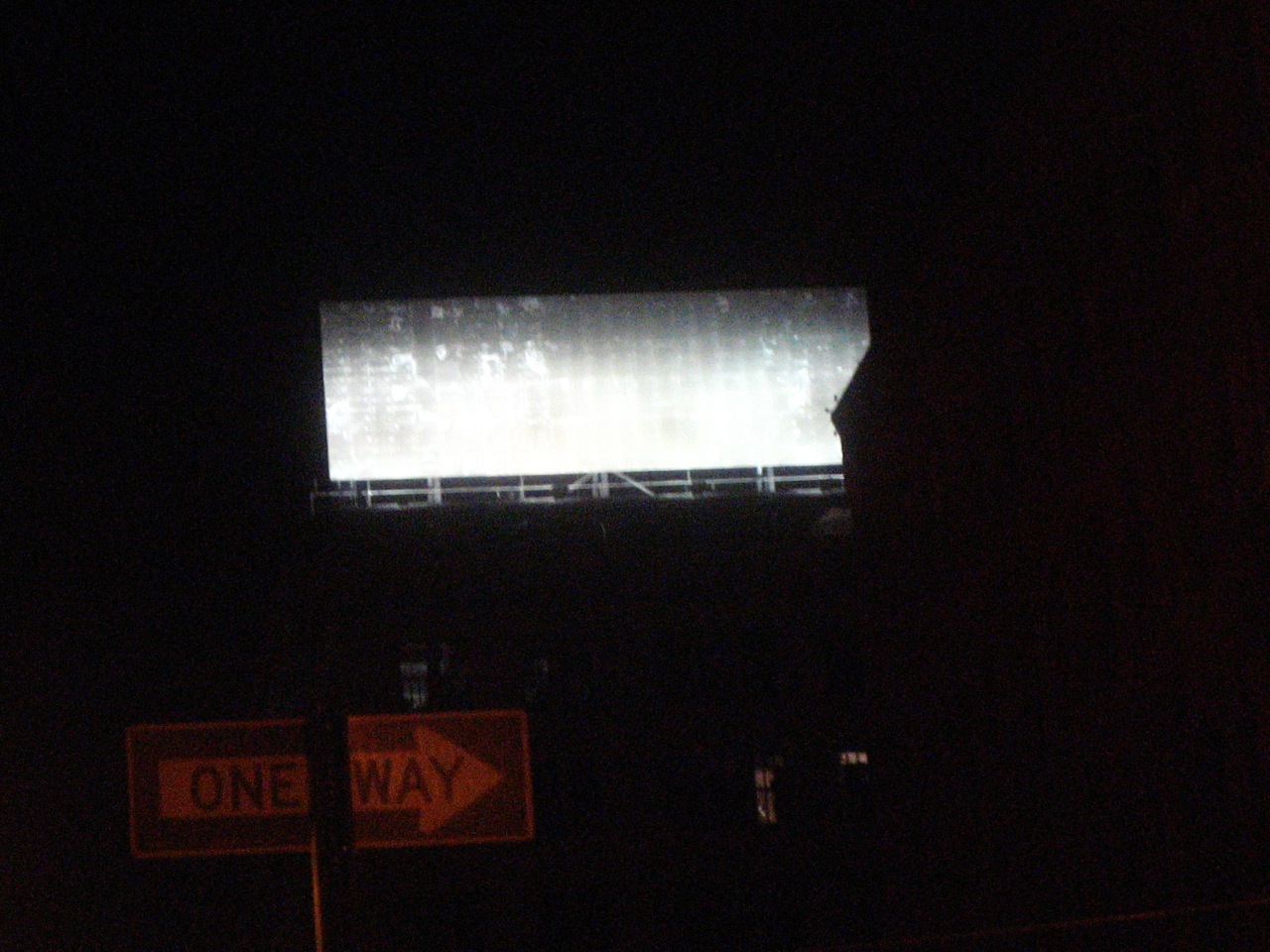In this dimly lit, nighttime photograph, a one-way highway sign prominently points to the right, guiding traffic in the intended direction. The scene features a large, illuminated billboard in the background, which, although brightly lit, displays no discernible text or images due to the distance and lighting conditions. The billboard appears to be situated near a fence, creating a sense of enclosure. Additionally, at the lower edge of the image, there are visible windows emitting warm light from within, suggesting occupied buildings nearby. The overall composition captures a solitary, nocturnal atmosphere with subtle urban elements.